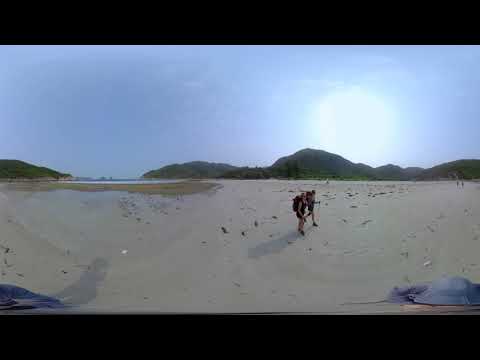The rectangular photograph, framed by black bars at the top and bottom, captures a vibrant beach scene under a clear blue sky. Dominating the background is a huge, bright sun that casts its glow over the sandy landscape. In the center, a man and a woman can be seen hiking, both donning shorts, tank tops, walking sticks, and large backpacks, indicating a warm, sunny day. They are slightly crouched, perhaps examining the ground, where scattered birds, rocks, or seashells are visible on the tan sand. Behind them, a lush, green mountain range runs horizontally across the scene with a smaller hill on the left side. There is also a hint of water in the far left background, adding to the serene atmosphere of the beach setting.